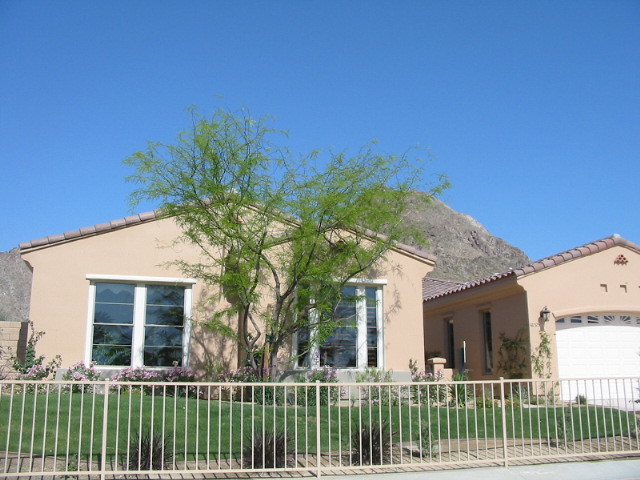The photograph depicts a suburban house set against a backdrop of a gray-colored rock formation or mountain. The house is beige with a light brown tiled roof, complemented by darker brown shingles or tiles. Large, rectangular windows with white frames dominate the front, and a white garage with windows is situated on the right side, seemingly detached from the house.

A beige-colored metal fence, featuring vertical bars, encloses the property, including a green lawn adorned with cut grass, small shrubs, and a medium-sized tree with green leaves. The front yard also features rose bushes in bloom with white and purple flowers. The left side of the garage displays some ivy growth.

The sky above is a clear, bright blue, occupying nearly half of the photograph, while the background reveals hills or mountain ranges with a mix of brown dirt and green grass. There's a gray brick wall to the left and gray bricks on the ground near the house. The image also captures a portion of the street on the bottom right corner.

The overall scene is a tranquil suburban setting, framed by natural elements and a crisp blue sky.